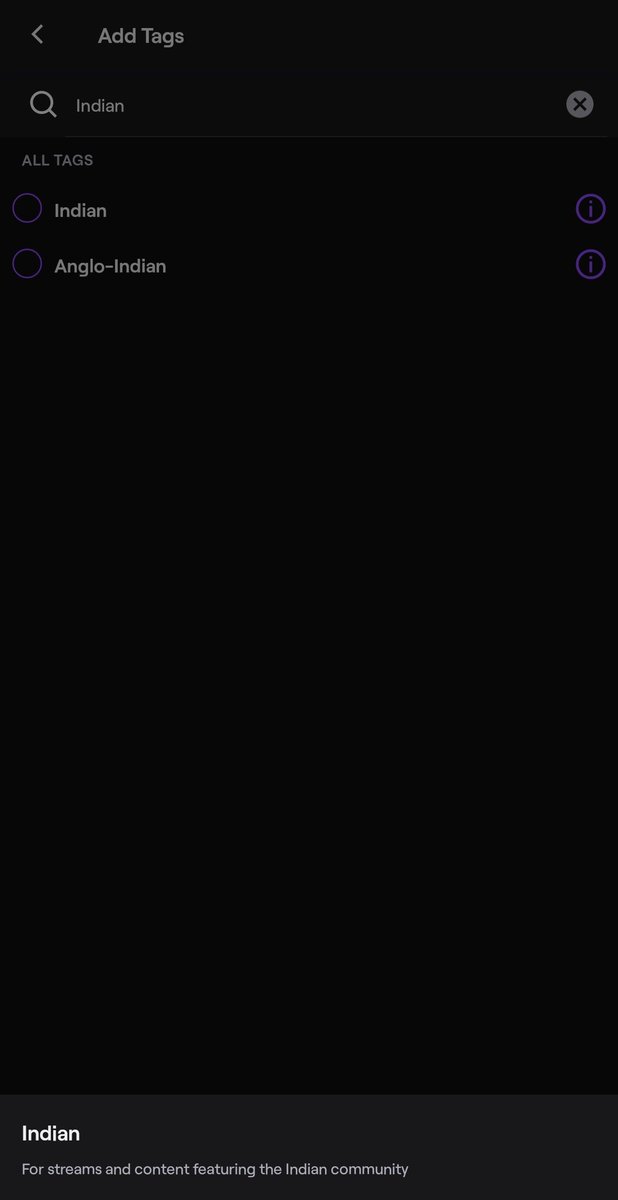Caption: 

On a black background with white text, the image features search results for streams and content highlighting the Indian community. Behind the text "Indian" is a gray backdrop. The terms "Indian" and "Anglo-Indian" both have circles next to them, indicating filter options. The tags include "Indian," "Anglo-Indian," and other related terms.

#Indian #AngloIndian #Community #CulturalContent #Streaming #ContentTags